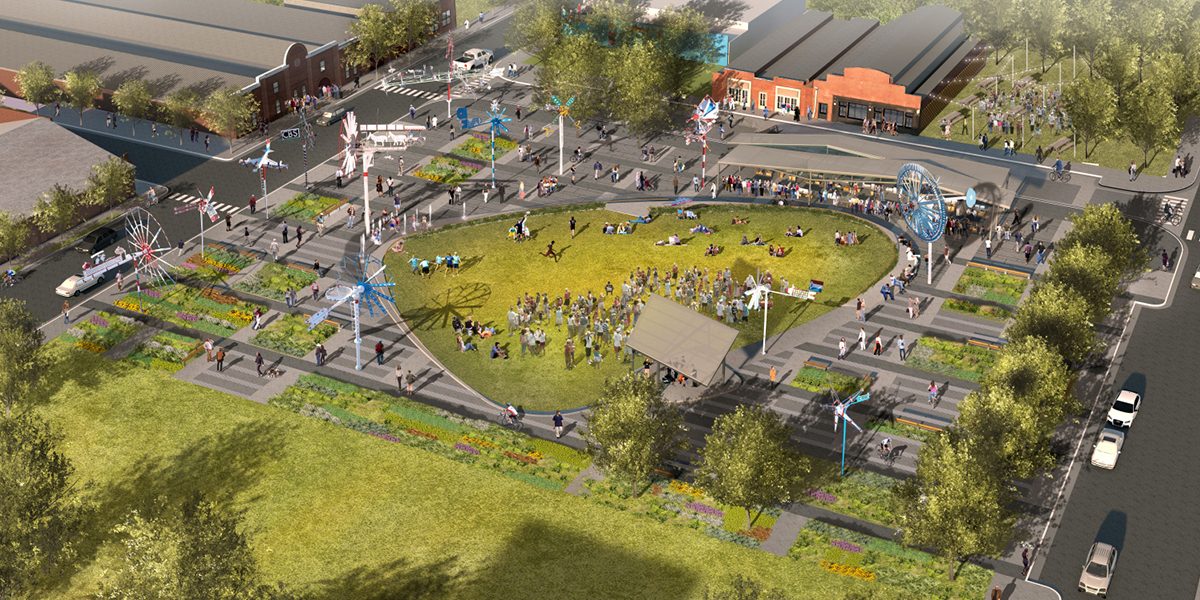This aerial view image captures a large, multi-purpose field that appears to serve as an equestrian event space. The grass field is somewhat heart-shaped and surrounded by an outdoor stadium with seating areas and lighting poles. In the center of the field, a crowd of people and their horses gather, indicating the event's focus on equestrian activities. Surrounding the field are various structures including a small house on one end and a Ferris wheel on the other end. There are also longer buildings that resemble airplane hangars, possibly hinting at an adjacent aerospace park or small municipal airport. To the left and right of the field are roadways with parked cars and a red, brick building with a multi-level roof, potentially a school or auditorium. The vicinity is adorned with numerous trees, adding a lush green backdrop to this multifaceted location.